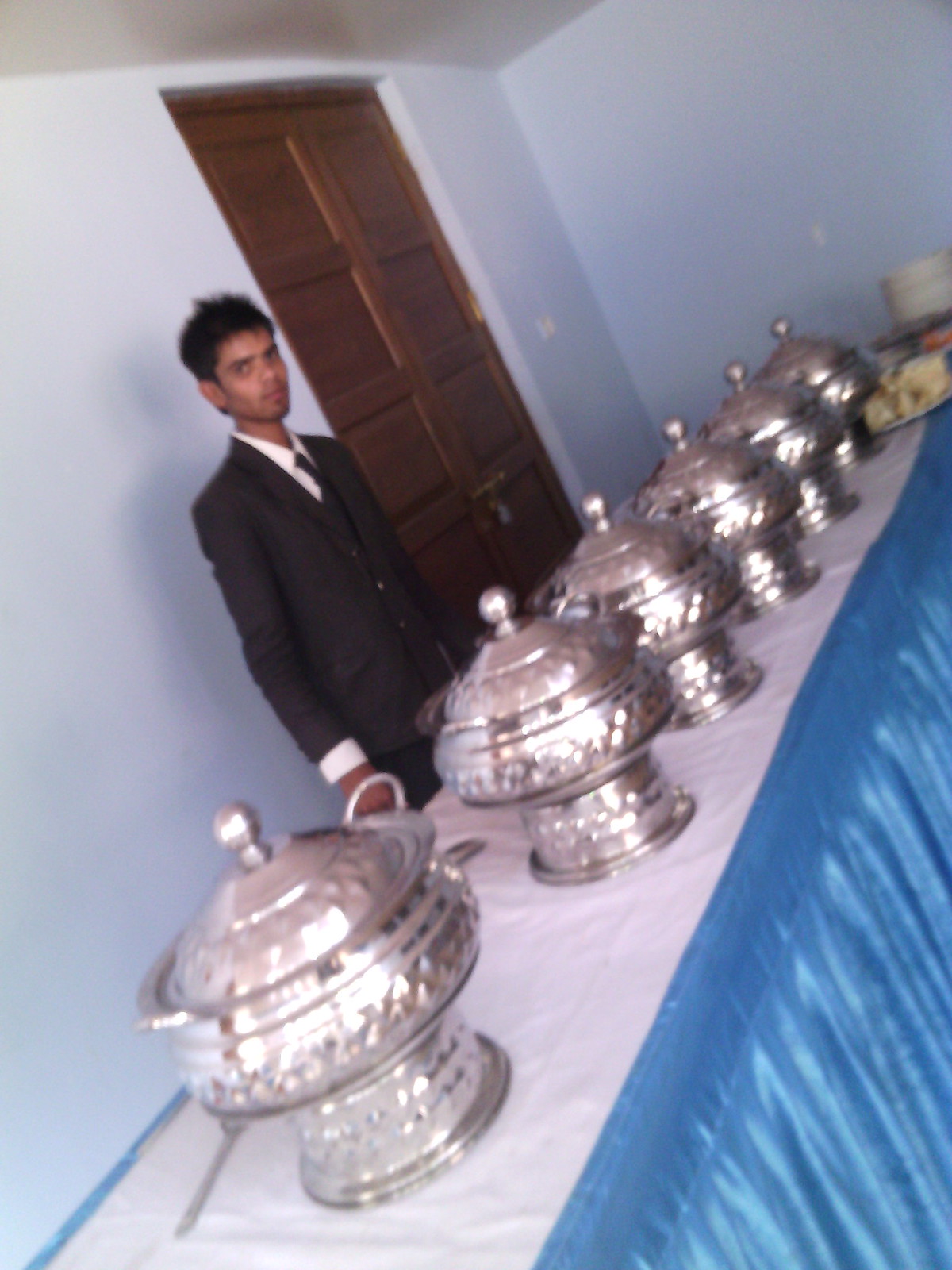In the slightly blurry photograph of a modestly decorated banquet or event, a man in a black suit and tie stands behind a long table, possibly in a serving role. The table, covered with a white tablecloth on top and a satin-like light blue cloth along the sides, displays six large, ornate, silver serving bowls with lids, arranged neatly in a row. At the end of the table, a plate of food and a stack of plates can be seen, suggesting that the buffet is not yet ready for guests to serve themselves.